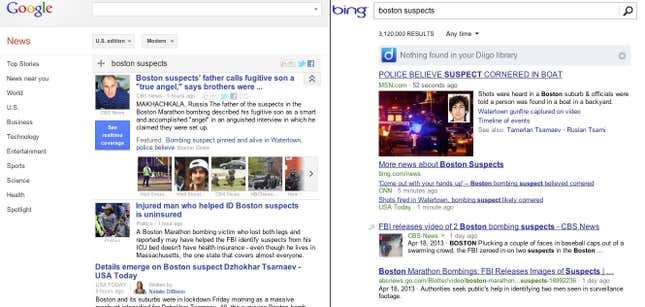The image compares search results from Google and Bing for the query "Boston Suspects." 

**Google Search:**
- The search query entered is "Boston Suspects."
- The first result is a news story titled "Father calls fugitive son a true angel, says brothers were..."
- The search includes a prominent image of a balding man, presumably one of the suspects.
- The results fall under the "News" category, with additional subcategories listed: "Top stories," "News near you," "World," "U.S.," "Business," "Technology," "Entertainment," "Sports," and "Science."

**Bing Search:**
- The search bar indicates that no relevant information was found in the "Diego Library."
- A visible link suggests police believe a suspect is cornered in a boat.
- The search results feature an image of a young man with dark hair in the top right corner, along with another obscure, dark outdoor scene that is difficult to discern.
- The Bing interface offers several categories to explore further information related to "Boston Suspects."

The comparison highlights the differences in how Google and Bing display and prioritize information, including the organization of news categories and visual elements such as images associated with the search query.